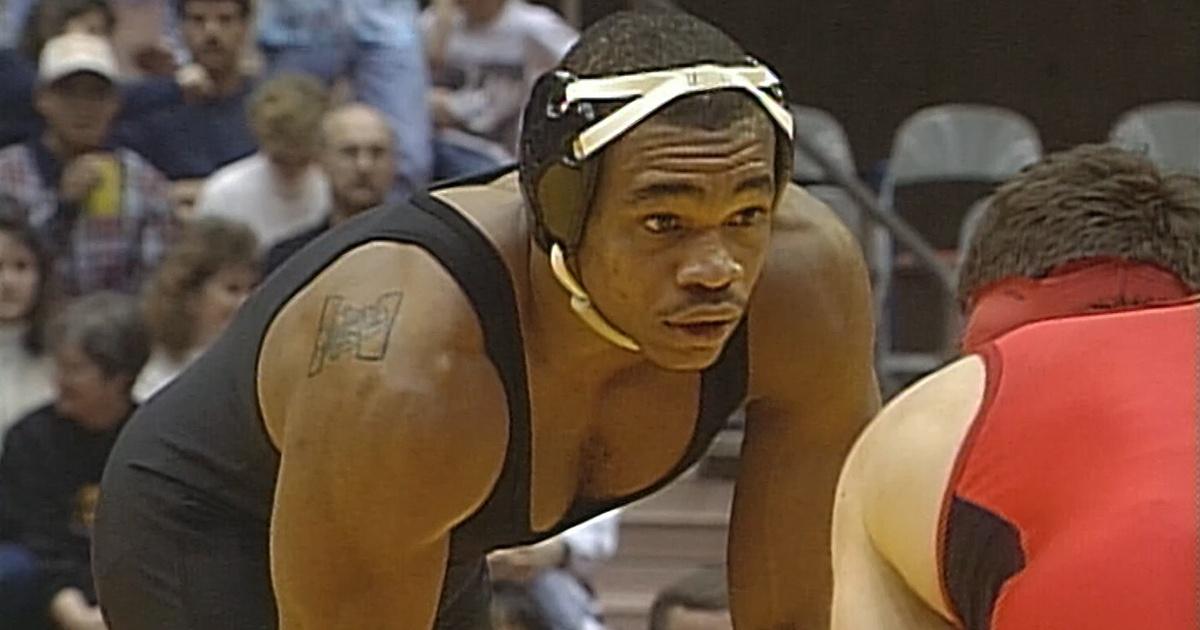In this detailed image, an African-American male wrestler, sporting a black sleeveless unitard and prominent black ear protectors with white straps crossing his forehead, is positioned centrally. His short buzz cut and a tattoo on his right shoulder are visible as he slouches forward, intensely facing his opponent. The opponent, seen only from the back, has lighter skin and wears a red sleeveless wrestling outfit with similar ear protectors. Both wrestlers are captured mid-match, leaning towards each other in a wrestling stance. In the background, an audience can be seen seated in the bleachers, attentively watching the unfolding match.